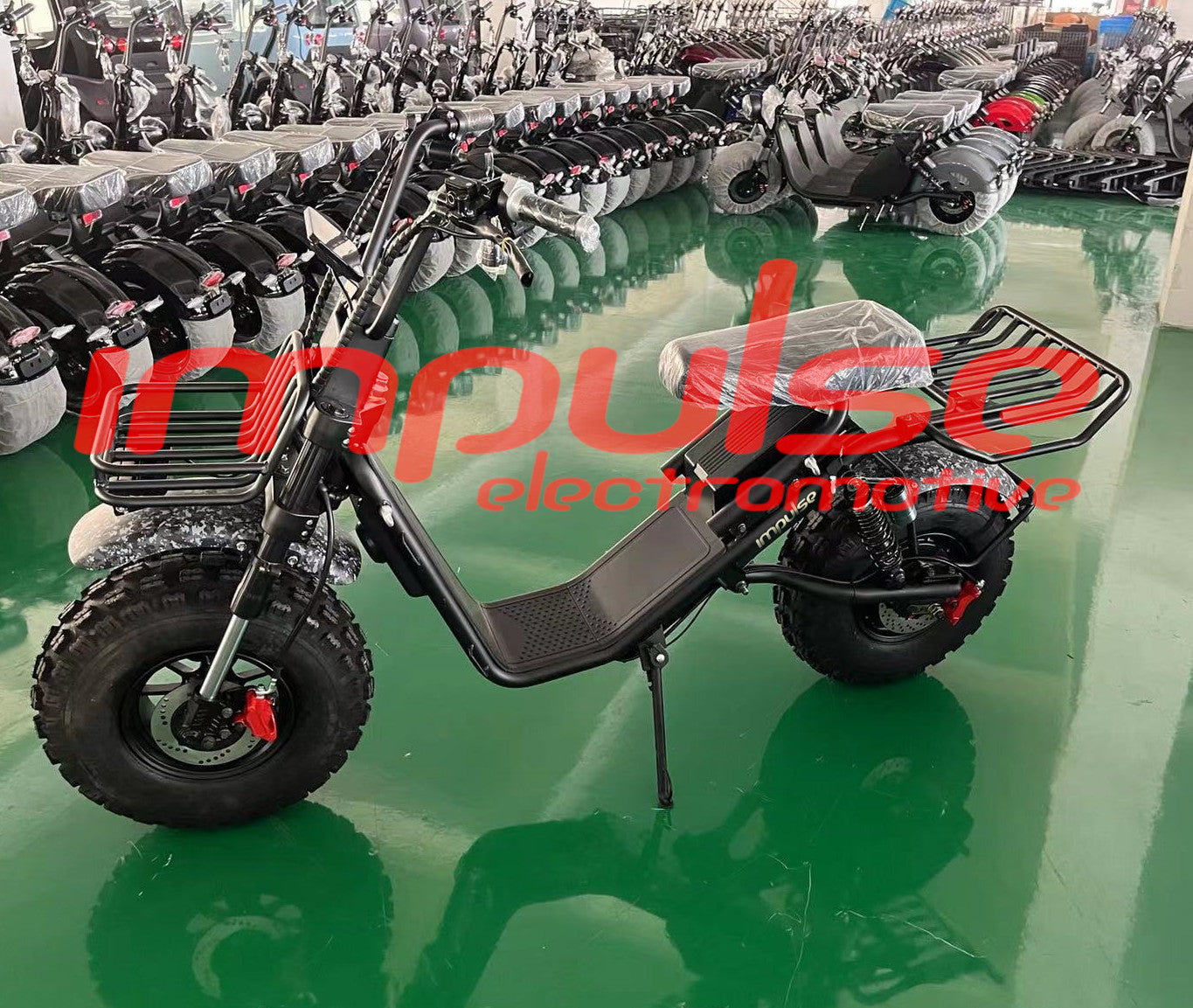The image showcases a showroom filled with sleek, black electric bikes branded as "Impulse Electro-Motive." These vehicles resemble a cross between mopeds and motorcycles, with two wheels and a kickstand for support. Each bike features a seat covered in plastic wrap, indicating they are brand new. The bikes are meticulously arranged on a highly reflective green floor, extending in rows that give the illusion of an endless array. Both the front and back of each bike are equipped with baskets, adding to their utility. The setting appears to be a warehouse or a store preparing these bikes for shipment or display, highlighting their modern design and abundance.